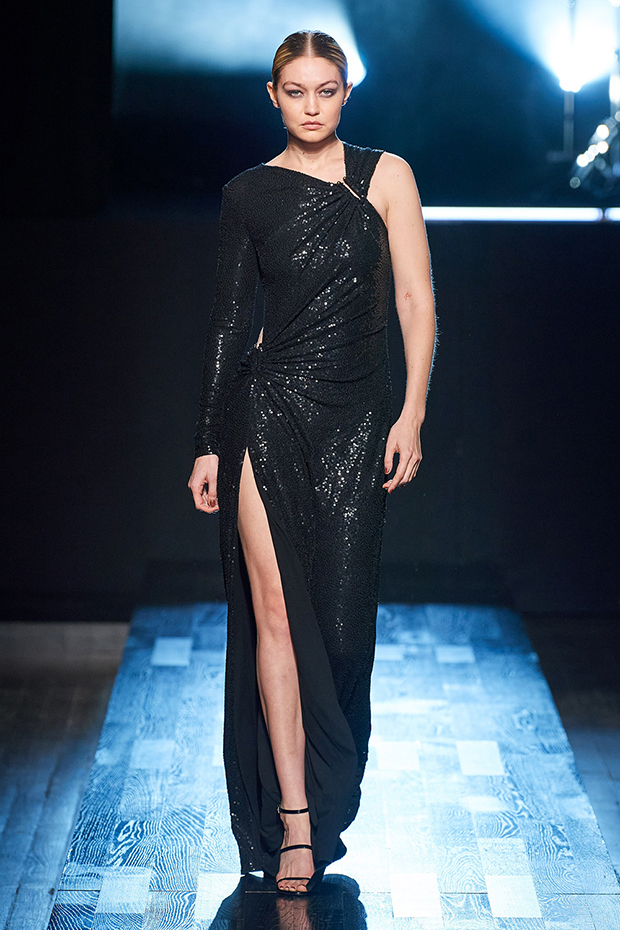The image is a professionally shot, full-color photograph set indoors under artificial light, showcasing a young Caucasian model confidently walking down a runway. The background is predominantly dark, with noticeable light sources in the upper right corner and behind her, creating a striking contrast. The model's serious expression and statuesque presence draw the viewer's focus directly to her.

She is wearing an elegant, full-length black dress with a striking design: the right side of the dress features a sleeveless strap, revealing her entire arm and shoulder, while the left side has a full sleeve. The right leg is prominently displayed through a high slit running up to about mid-thigh, adding a bold touch to the outfit. She is also wearing black heels, which are partially visible due to her forward stride.

Her hair, a mix of brown and dirty blonde shades, is parted in the middle and pulled back, possibly into a bun or ponytail. The runway itself seems to be made of wooden slats with a polished sheen and a blue cast, likely from the surrounding lights, enhancing the overall moody and sophisticated atmosphere of the scene.